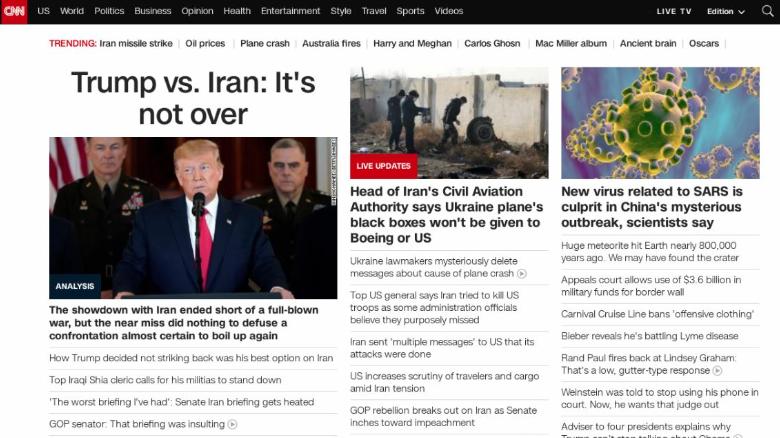This screen capture of the CNN website prominently features its familiar branding and navigational elements at the top. The well-known red square with the white CNN logo is positioned in the left-hand corner. A horizontal black bar spans the width of the page, displaying the menu in white lettering; categories include U.S., World, Politics, Business, Opinion, Health, Entertainment, Style, Travel, Sports, and Videos. On the far right, this bar lists "Live TV," followed by "Edition" with a down arrow, and a white search glass icon.

The main story is headlined in bold black lettering: "Trump versus Iran: It's not over." Below the headline, a photograph depicts President Trump during his tenure, flanked by military personnel on either side. Trump, notably, is wearing a red tie. The accompanying text describes how the showdown with Iran ended short of a full-blown war but did not diffuse tensions, which are likely to escalate.

Central to the page, another headline reads: "Head of Iran's Civil Aviation Authority says Ukraine plane's black boxes won't be given to Boeing or U.S." The image above this headline shows military personnel seemingly searching through rubble. A red banner in the lower left corner of this image reads "Live Updates" in white lettering.

To the right, another headline states: "New Virus Related to SARS is Culprit in China's Mysterious Outbreak, scientists say." This is accompanied by an image displaying the molecular structure of the COVID-19 virus.

Each photograph is accompanied by lengthy additional listings of articles. Above the "Trump versus Iran" headline, the word "Trending" appears in red text, indicating the popularity of the article.